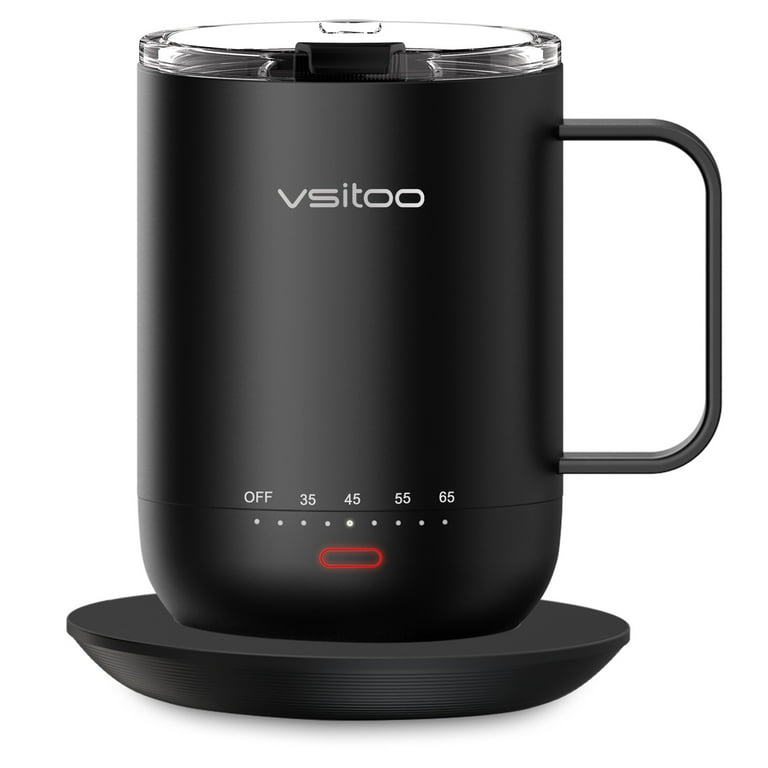The image features a sleek, matte black electric heated mug branded with "VSITOO" on its left side. The mug, which has a sharply angled rectangular handle, stands on a matching black heating pad. The lid of the mug is clear plastic with a black locking mechanism over the drinking area. Below the mug, a red oval button likely functions as the power indicator. An adjustable temperature control, which includes settings of 35, 45, 55, and 65 degrees, is situated near the bottom of the mug. The setup appears compact and modern, ideal for keeping beverages warm. The white background highlights the mug's elegant design and functionality.